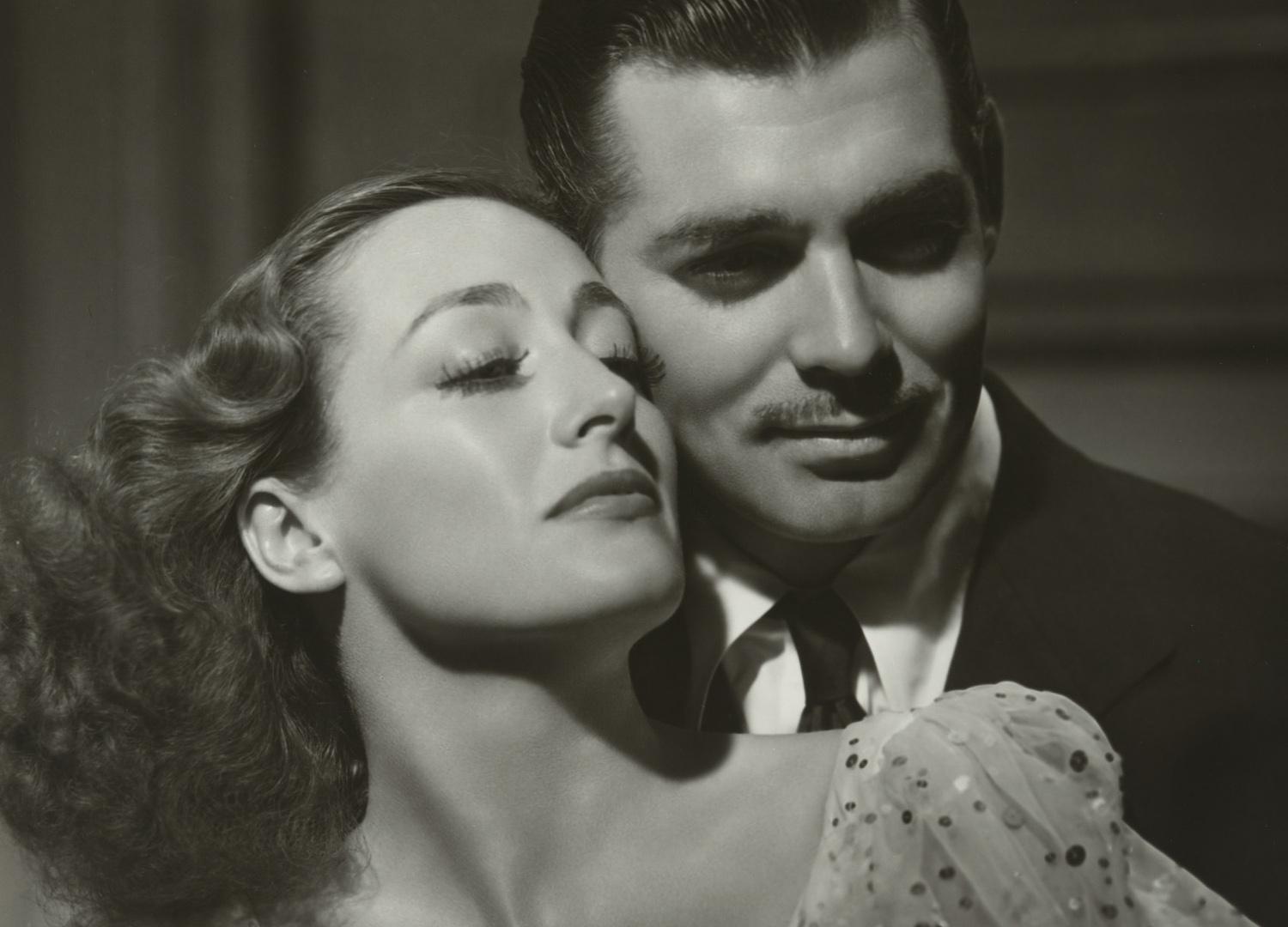This black-and-white still from a classic movie features a handsome man with slicked-back dark hair and a pencil mustache, dressed impeccably in a dark suit, white button-down shirt, and dark tie. He stands in the background, smiling subtly, with his body partially facing forward but his head turned slightly to the right. A charming woman, positioned in the foreground to his left, has voluminous, wavy dark hair and strikingly long eyelashes. She wears an elegant, light-colored, sequined dress with poofy, lacy shoulders, exuding an air of sophistication. Their faces almost touch, suggesting an intimate moment, possibly mid-dance. The background is blurred, with indistinct vertical lines indicating a wall or room, further focusing attention on the pair's nostalgic grace and charm.